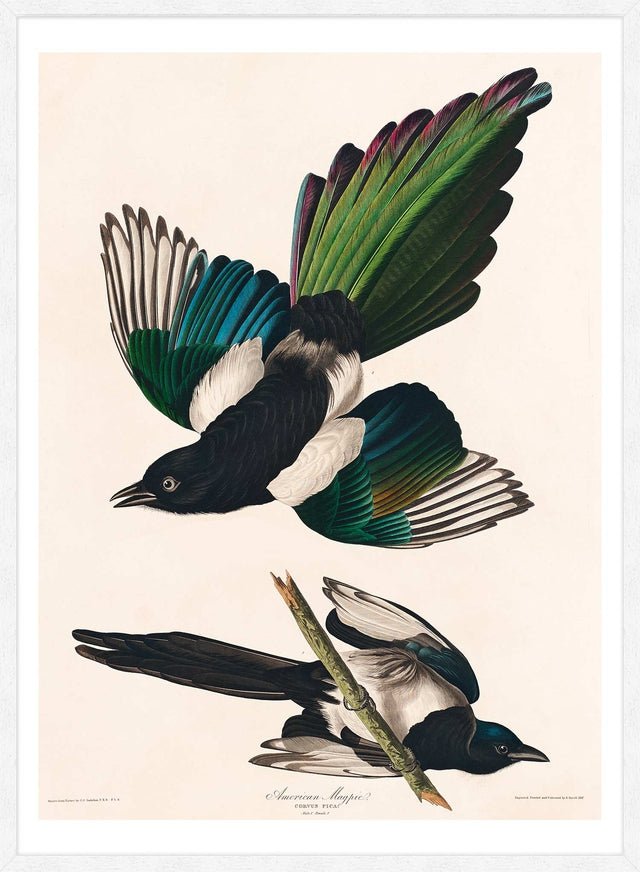The framed artwork features a light off-white background and includes two detailed illustrations of an American magpie, identified by cursive text at the bottom of the frame. The upper illustration depicts the magpie flying downwards, showcasing its vibrant wings and tail. The tail feathers are predominantly green with red or pink accents, while the wings exhibit a gradient from green at the top, transitioning through blue, and ending in white with slight orange highlights. The bird's head and upper body are black, reminiscent of a crow, with distinguishable white feathers interspersed between the wings and body. The magpie's beak is slightly open, and its eyes feature a striking white and black pattern.

In the lower illustration, the magpie is portrayed from a different perspective, sitting on a greenish-brown branch, with its underbelly and underside of the tail visible. The underbelly and the bottom of the wings are primarily white, while the under tail feathers are black. The head and neck maintain the same black coloration as seen in the top illustration, emphasizing the bird's distinctive markings. Additionally, there is small, somewhat hard-to-read text in the bottom left and right corners of the image, suggesting it might serve as a reference or identification guide for birds.